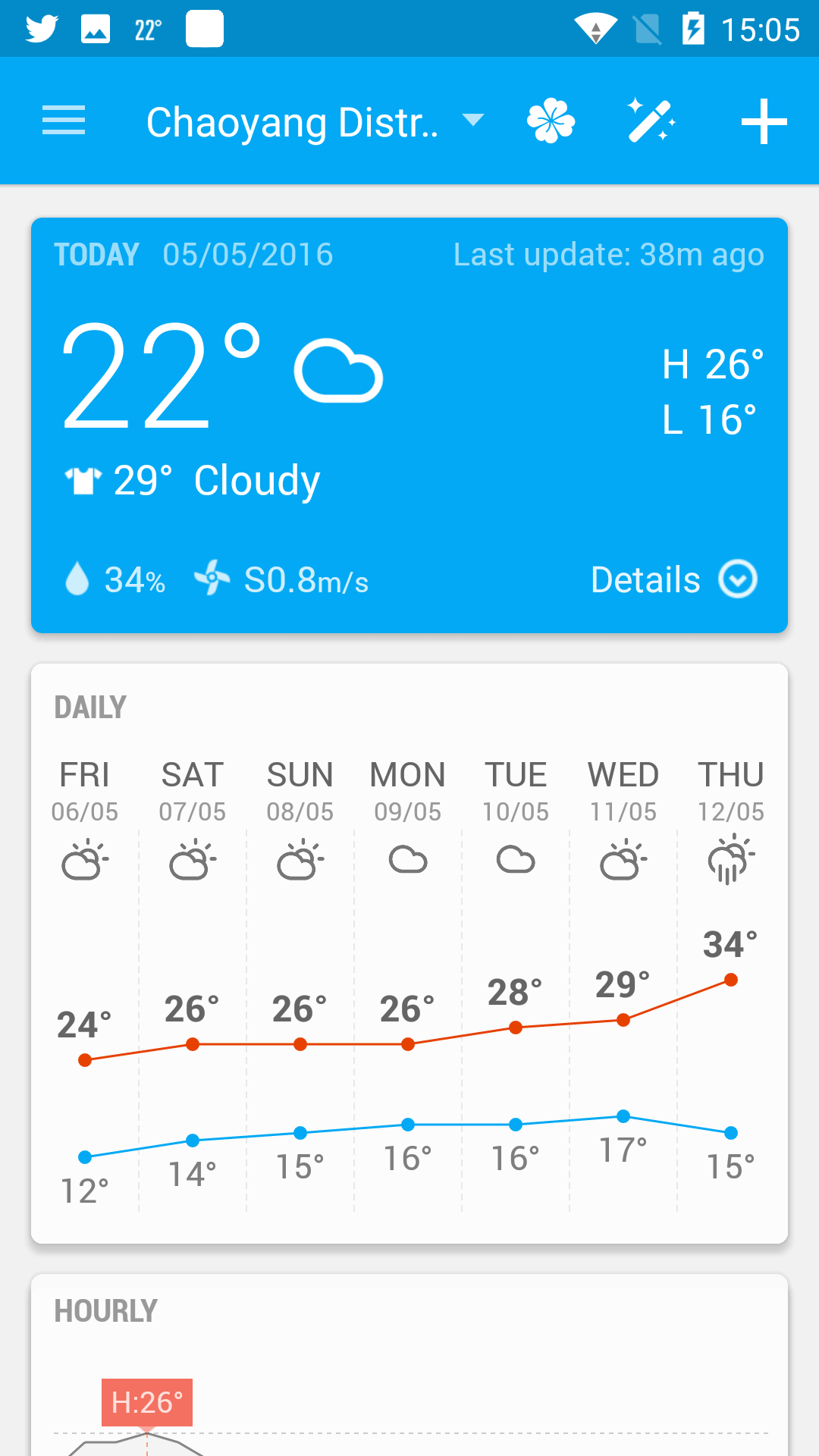Screenshot of a weather app on a smartphone displaying detailed weather information for Chaoyang District, China. The interface features a blue header with icons for Twitter, a photo gallery, Wi-Fi, and a battery meter, along with the current time of 15:05. The location "Chaoyang District" is highlighted in a lighter electric blue header, accompanied by icons including a four-leaf clover, a pen with sparkles, and a plus sign. 

The main panel is divided into three sections:

1. **Current Weather**: A blue bar displaying the date (05-05-2016) and a last updated timestamp (32 minutes ago). The current temperature is 22°C, indicated by a cloud icon. Additional details show 29°C and cloudy, 34% humidity (indicated by a water drop icon), and wind speed coming from the south at 0.8 meters per second, represented by a pinwheel icon. The high is 26°C and the low is 16°C, with more detail options available below this section.

2. **Weekly Forecast**: A white panel presenting the forecast for the coming seven days:
   - Friday: Cloudy, High 24°C, Low 12°C
   - Saturday: Cloudy, High 26°C, Low 14°C
   - Sunday: Partly Cloudy, High 26°C, Low 15°C
   - Monday: Cloudy, High 26°C, Low 16°C
   - Tuesday: Cloudy, High 28°C, Low 16°C
   - Wednesday: Cloudy, High 29°C, Low 17°C
   - Thursday: Rainy, High 34°C, Low 15°C

   Each daily forecast is accompanied by a red and blue line graph indicating the temperature trends.

3. **Hourly Forecast**: A section at the bottom of the screen, not fully visible in the screenshot.

This detailed view provides comprehensive, up-to-date weather information to keep users informed about current conditions and upcoming forecasts in Chaoyang District.